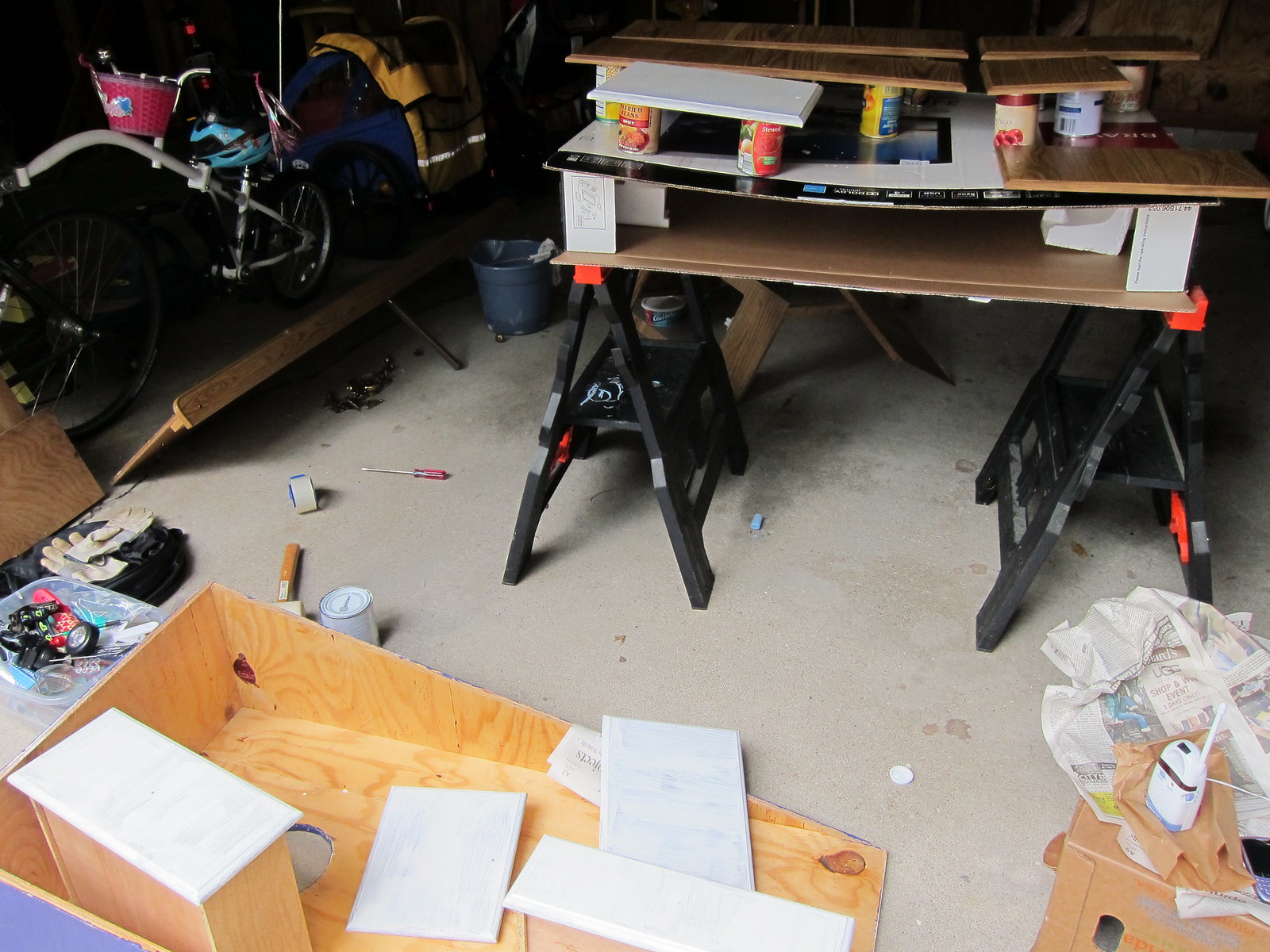The image depicts the interior of a multi-purpose space that combines elements of a workshop and a storage area, likely within someone's garage. The setting features a concrete floor laden with various items, including makeshift metal stands supporting several wooden planks, suggesting ongoing woodworking or furniture construction. Among these, wooden cabinets and detached cabinet doors are visible, some of which are supported by cans and other readily available items. A partially disassembled wooden cabinet is situated prominently on the floor, with its drawers painted white, hinting at possible refinishing or restoration work. To the left, a bicycle adorned with a pink basket is parked, surrounded by an assortment of miscellaneous items, contributing to the scene's organized yet cluttered atmosphere.